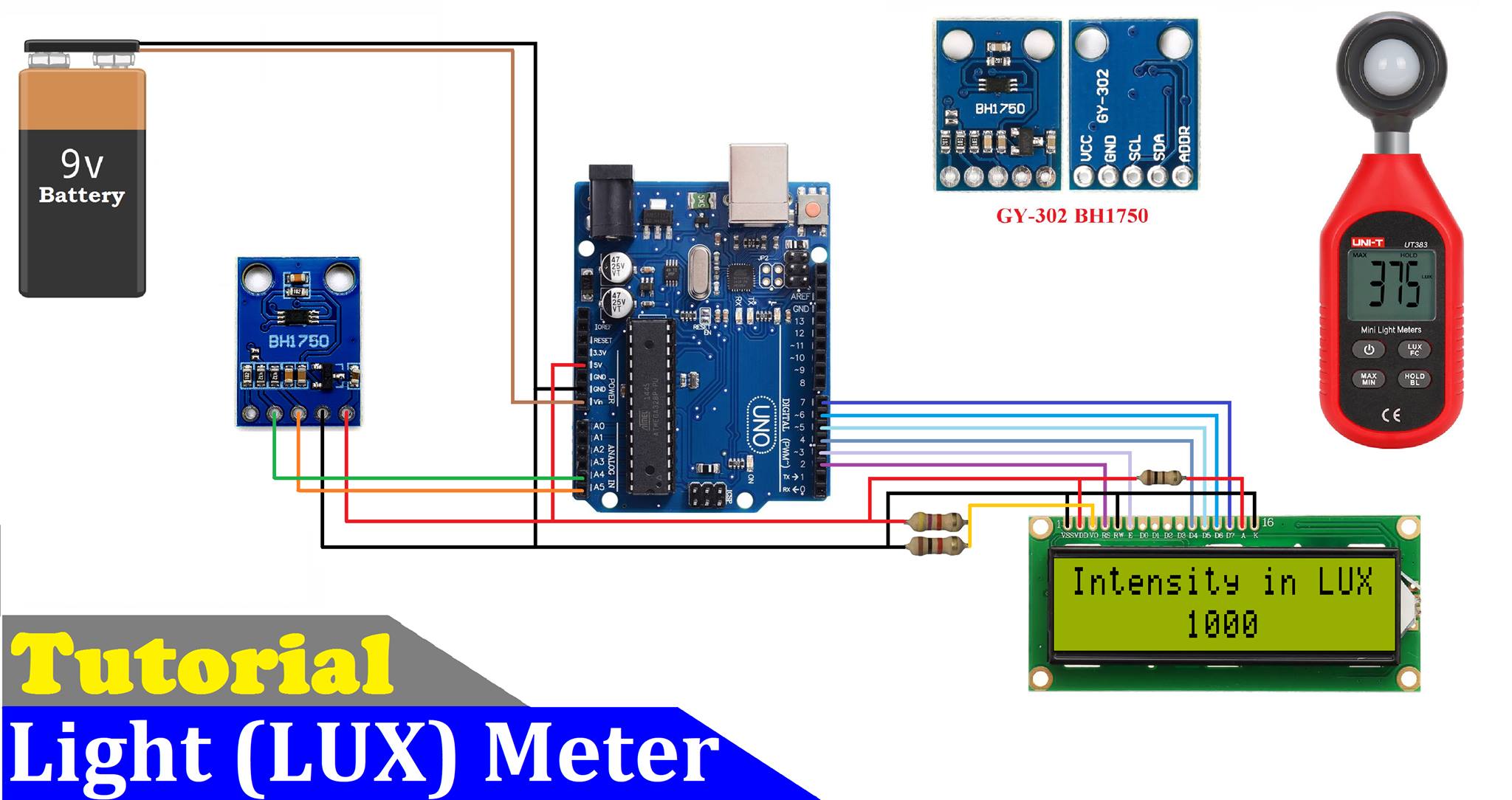The image displays a detailed module system used to assemble an amateur-built light meter. On the left side, there is a 9-volt battery resembling a Duracell, characterized by a brown top and black bottom. Next to it, a label reads "Tutorial Light Lux Meter" against a gray background with yellow text. 

In the center of the image, there is a blue electronic circuit board featuring various black components. To the left of this board, a blue sensor labeled BH1750 is present, linking the battery and the central circuit board. Additionally, below this setup, the phrase "Intensity Lux 1000" can be seen, indicating part of the light measurement system.

On the right side of the image, a red handheld light meter with a black display screen is prominently shown, displaying the number 375. This device has a distinctive black section in the center and is fitted with a white spherical light sensor mounted on a metallic rod at its top. This setup is intended to measure light intensity, utilizing components such as a microcontroller to read the data.

Conclusively, this diagram illustrates the interconnections between the battery, circuit boards, and sensors, showing the flow of power and data within the light meter system.